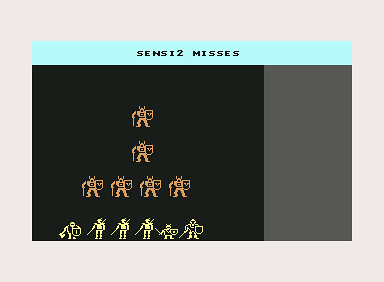This image appears to be a still from a video game, showcasing gameplay elements and on-screen text. At the very top of the screen, there is small black text that reads "S-E-N-S-I-2 MISSES" on a long, light blue rectangle. Below this, about one-fourth of the right area is dark gray, while the remaining area is black.

The gameplay scene is arranged in rows:
- The top row features a small orange character, less than an inch tall, with little lines above its head. The character seems to be holding a square object, possibly a computer or a similar device.
- The second row mirrors the top row, displaying another small orange character holding a square object.
- The third row includes four of these small orange characters, each maintaining the same design characteristics.
- The bottom row showcases characters in yellow hues. There appears to be one character holding a shield and three others holding swords. Among these, one character wields a short sword along with a shield, and the final character also holds both a sword and a shield.

The arrangement hints at a formation or lineup, likely indicative of a team or group preparing for an objective or battle within the game.